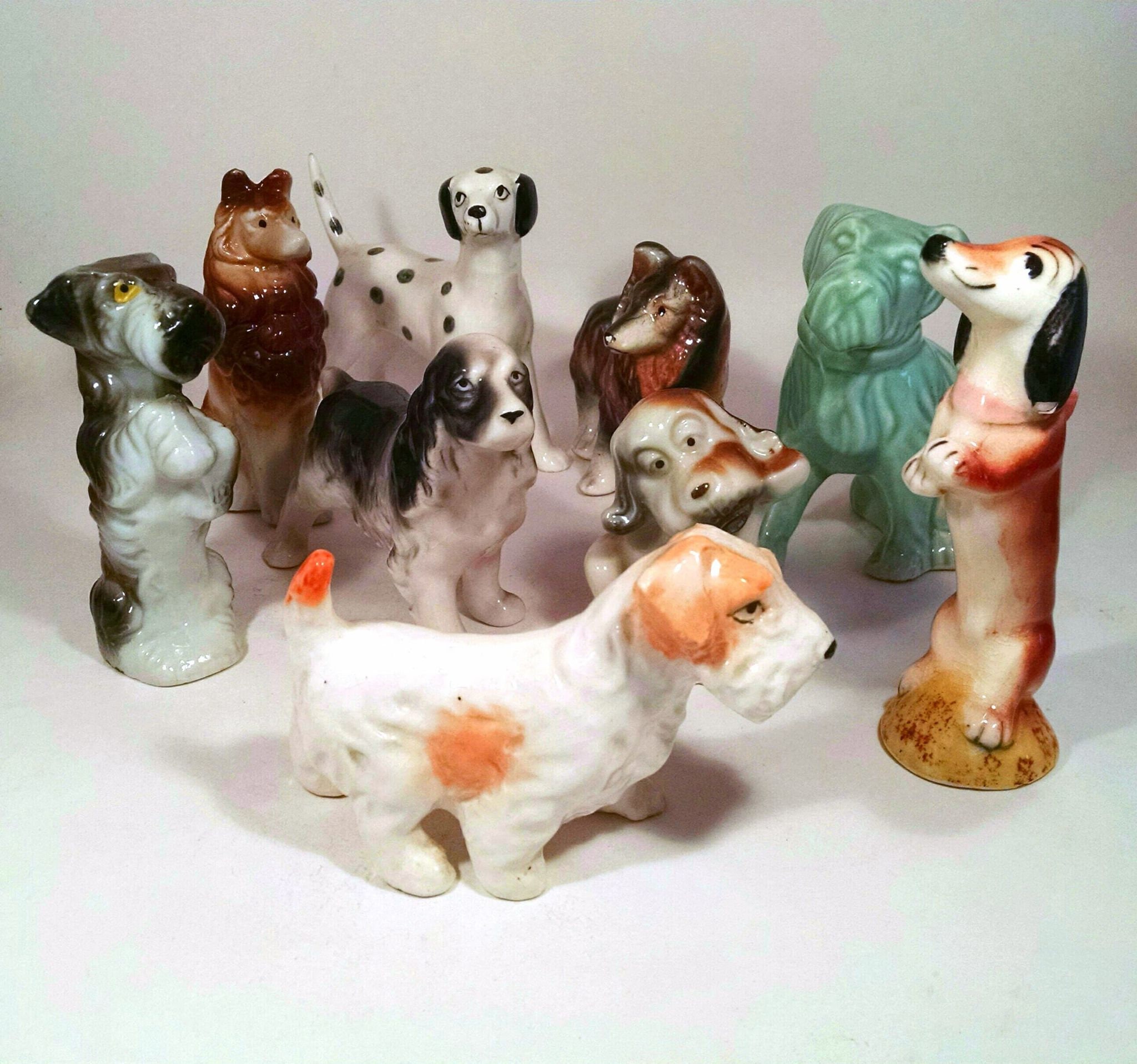The image displays a collection of nine detailed dog figurines arranged on a white background. These figurines appear to be made from either glass or porcelain. Each dog is unique in its breed and coloring, contributing to the diversity of the collection. 

Prominently, there is a white dog with brown patches and an orange-tipped tail in the front. To the left side, a white dog with a black head and back stands on its hind legs. A brown wolf-like dog is positioned next to this figurine, while a Dalmatian with distinctive black spots and black ears stands towards the back. Near the Dalmatian is another dog with a white body and black top and ears.

Further adding to the variety, another brown, wolf-like dog stands on all fours next to a mint-green colored dog in a sitting position. There's also a small dog that resembles a sausage dog with a white undercarriage, light brown back, and black ears, sitting on its hind legs. Centrally, a white dog with a face divided in color - brown on one side and black on the other - has its head tilted to the side, offering an endearing look.

Each figurine is meticulously crafted, featuring an array of colors such as brown, white, black, and even green, highlighting the individual characteristics of different dog breeds including a Dalmatian, Doberman, Maltese, and Border Collie among others.